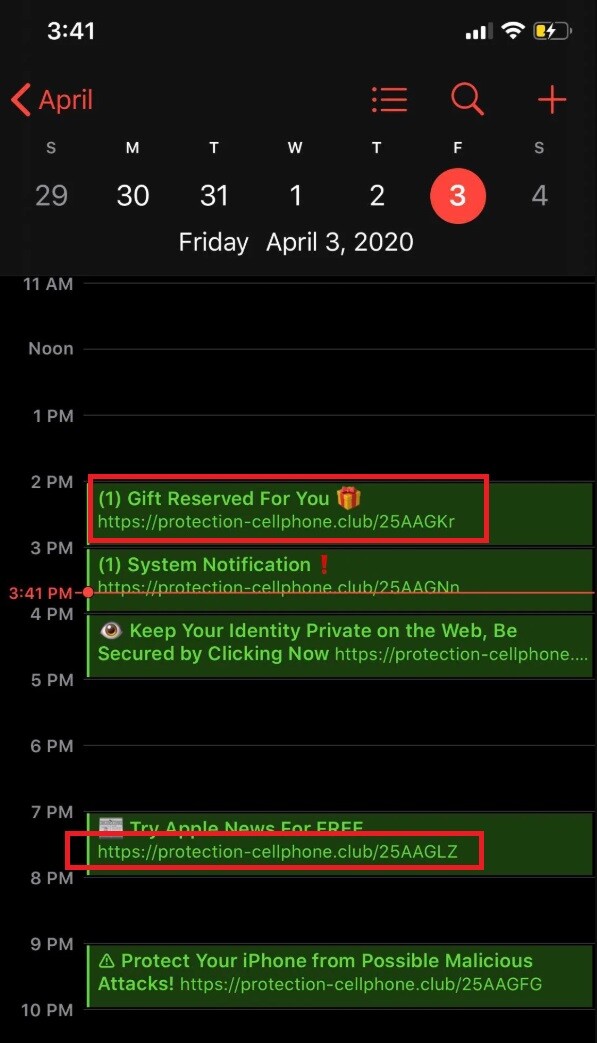The next image is a screenshot from a smartphone, displaying detailed information. In the top left corner, the time is shown as 3:41. On the far right, the Wi-Fi signal indicator shows three bars, suggesting a strong connection. The battery icon, located next to the Wi-Fi indicator, has a white lightning bolt in the center, indicating that the device is currently charging. The battery level is in the yellow zone, signifying that it needs charging.

Scrolling down, the month of April is displayed with a red arrow pointing left, likely indicating navigation options. Below this, the days of the week are shown in abbreviation: S, M, T, W, T, F, S, representing Sunday through Saturday. The specific date highlighted is Friday, April 3rd.

Further down on the calendar, the schedule starts at 11:00 a.m., which is empty. The subsequent hours are displayed as follows:
- 12:00 p.m. – No appointments or events.
- 1:00 p.m. – No appointments or events.
- 2:00 p.m. – A scheduled event titled "Number One and Gift Reserve for You." This entry includes a URL: smttfs://protection-cellphone.club/25AAGKR.

The final time displayed is 3:41 p.m., matching the current time shown at the top of the screen.